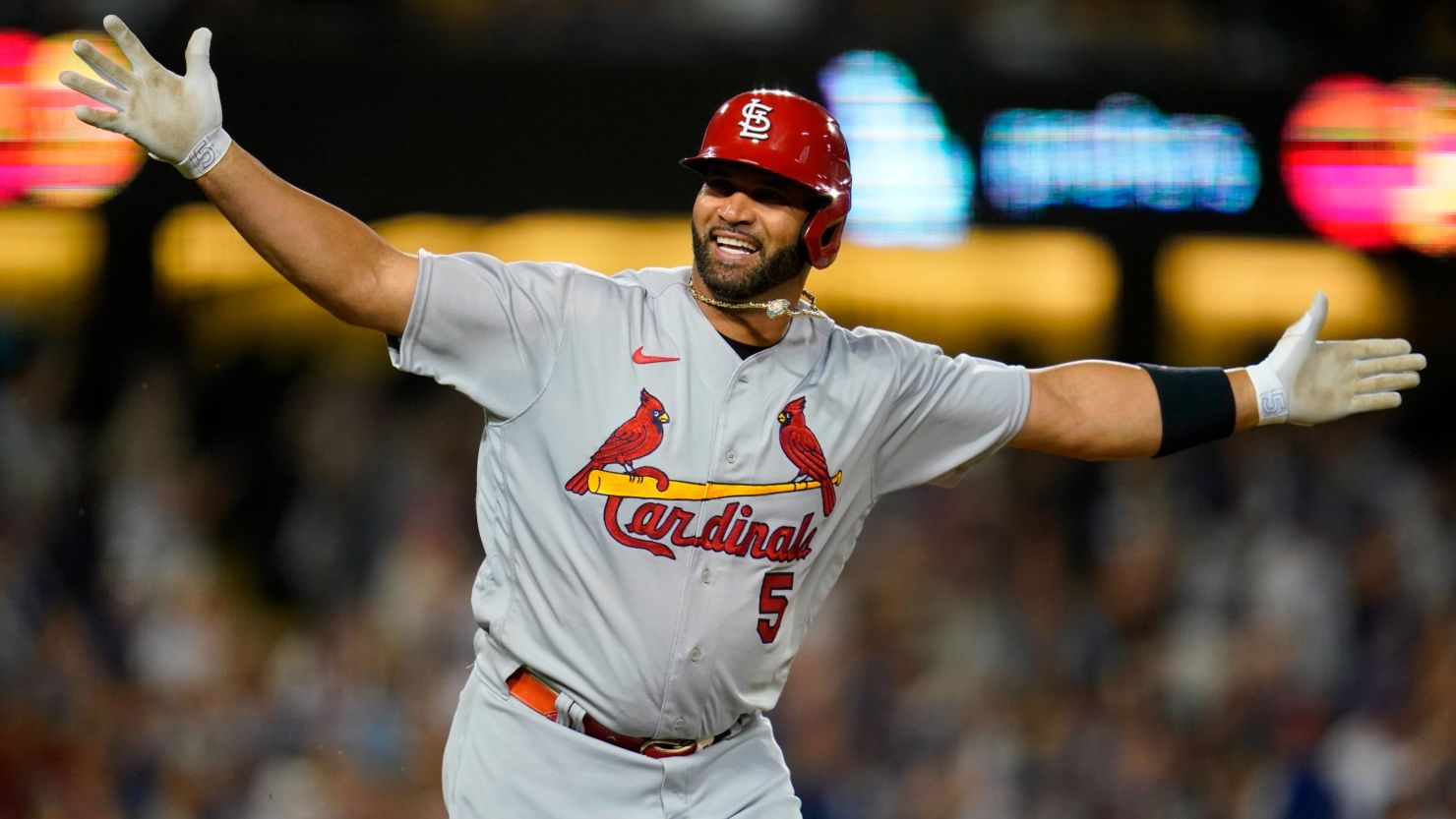The image displays Albert Pujols, the former baseball player renowned for his time with the St. Louis Cardinals. He stands central in the frame, striking a celebratory pose with his arms outstretched and his palms open, while flashing a wide smile and looking to the left. Pujols is a light-skinned black man with a black beard, donning a gold chain necklace. He wears a red batting helmet featuring the white "SL" Cardinals logo, along with a gray Cardinals jersey emblazoned with "Cardinals" in red text, the number 5, and a graphic of two red cardinals perched on a yellow bat. The jersey also sports a red Nike swoosh. His uniform is completed with gray pants, an orange belt, and white gloves that appear soiled. He also wears a black wristband on his left forearm.

The background consists of a blurred crowd of spectators in the stands, along with numerous lights, some blue and red. There's also additional blurred signage present on the upper left and right corners, with the upper left displaying a Visa or MasterCard logo. The overall ambiance conveys the energy of a live game, capturing Pujols in a moment of joy and triumph.